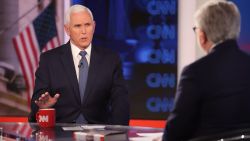This image appears to be a still shot from CNN, showcasing a television interview setup. In the background, the familiar CNN logo is prominently displayed on the wall multiple times and an American flag is visible, adding a patriotic touch to the scene. In the middle ground, former Vice President Mike Pence is seated at a glass table, engaging in conversation with an unseen interviewer whose back and shoulders are visible in the foreground. Pence, a Caucasian man with white hair and fair skin, is dressed in a black suit, white shirt, and blue tie, and he has one hand raised while speaking, his mouth open mid-sentence. A red mug featuring the CNN logo in white lettering sits conspicuously on the table in front of him. The interviewer, also wearing a suit and sporting grey hair, is turned towards Pence, creating an engaged and dynamic interview atmosphere.